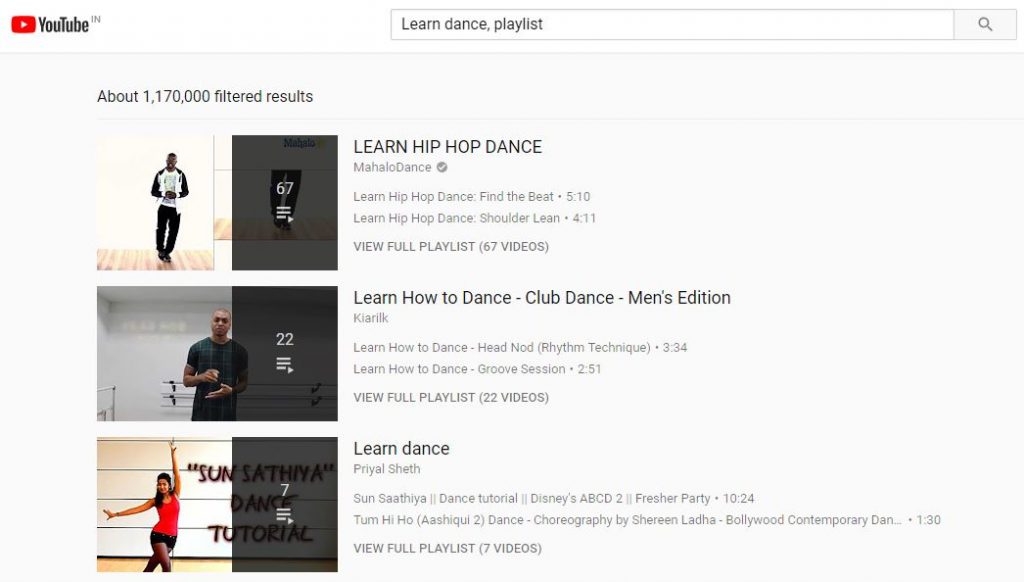This is a detailed screenshot of YouTube's search results page, featuring a search for "learn dance playlist." The background of the page is a light blue to bluish-gray gradient, with a white border at the top. In the top left corner of this white border, there’s a red square representing the Google Play button. To the right of this button, in bold black text, is the YouTube logo. 

Positioned just left of center, extending to the right, is the search bar with the text "learn dance playlist" in black inside it. To the right of the search bar is a small light blue square containing a black search icon. Below the search bar, the light blue background continues, and near the top, on the left side, there is a small inch-wide gap. Just below this gap, text indicates there are approximately "1,170,000 filtered results."

The main section displays three results for the search query. Each result features a preview image of dancing people. The first preview image shows a male dancer, the second also features a male dancer, and the third shows a female dancer. Each preview image is split into two sections: the left half is brightly visible, and the right half is overlapped by a black shadowy area with white-centered numbers indicating the video's duration. Below these numbers are three horizontal lines.

To the right of each preview image, the video titles are displayed in bold text. The first video is titled "Learn Hip Hop Dance," the second one is "Learn How to Dance – Club Dance – Men’s Edition," and the third is simply titled "Learn Dance." Under each video title is the name of the creator, followed by two lines of additional information about the video. On the far right, the video duration is listed. 

Below each video’s details, there is a link labeled "View Full Playlist," with the total number of videos in the playlist listed in parentheses. Each result is formatted in a similar layout, providing a consistent and organized display for the user.